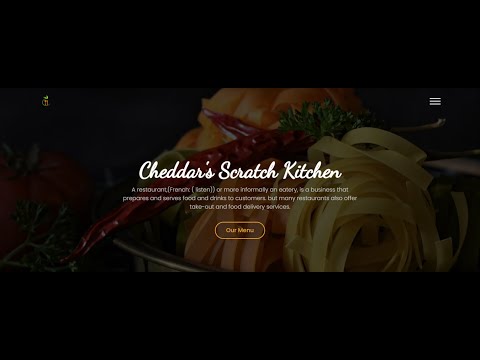This is a detailed and well-formulated caption for the described web page image:

"The web page for Cheddar's Scratch Kitchen features a striking, full-width photograph of a dish with noodles and a long red pepper, set against a black background. The image is centered, with black borders above and below. Prominently displayed at the center of the image is the name of the restaurant, 'Cheddar's Scratch Kitchen,' written in the largest font on the page. The text is in an italic, forward-slanting font that simulates a neat, hand-written style with elegant loops. Beneath the restaurant name, three lines of centrally aligned text provide additional information about the establishment. Below this text, there is a clickable box outlined in pale orange or cream color, containing the words 'Our Menu' in the same hue. While the food in the background is somewhat subdued compared to the vibrant central text, the tantalizing glimpse of the dish adds to the allure of the dining experience awaiting visitors."